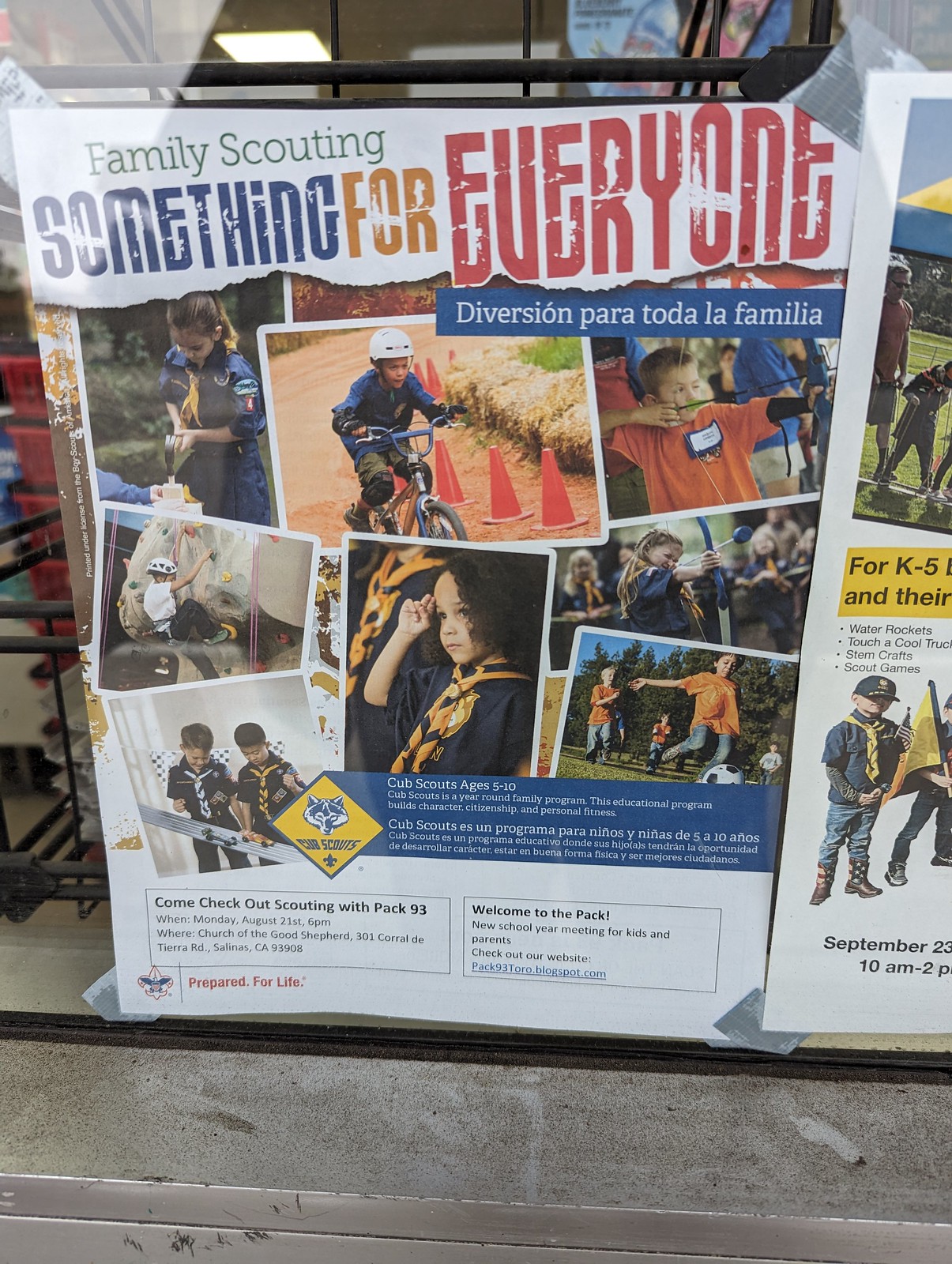This is a vibrant color photograph of a flyer displayed behind a glass window, likely of a storefront. The flyer, promoting family scouting, is filled with dynamic imagery and text both in English and Spanish. The top of the flyer prominently reads, "Family Scouting: Something for Everyone" followed by the Spanish translation, "Diversión para toda la familia." Below the text, several overlapping images capture young children engaged in various scouting activities. One child is seen riding a mountain bike through an obstacle course marked by orange cones, while another boy practices archery with a bow and arrow. There's also a child rock climbing and several boys and girls in blue and gold scouting uniforms, observing different activities. Another image shows children in blue jeans and orange t-shirts playing soccer. The bottom of the flyer contains fine print that invites readers to check out scouting with PAC 93, potentially including contact information in very small text. The poster's bright palette includes blue, red, orange, yellow, black, and tan, contributing to its eye-catching appeal. The overall layout features the images spread randomly across the flyer, capturing a sense of excitement and action.